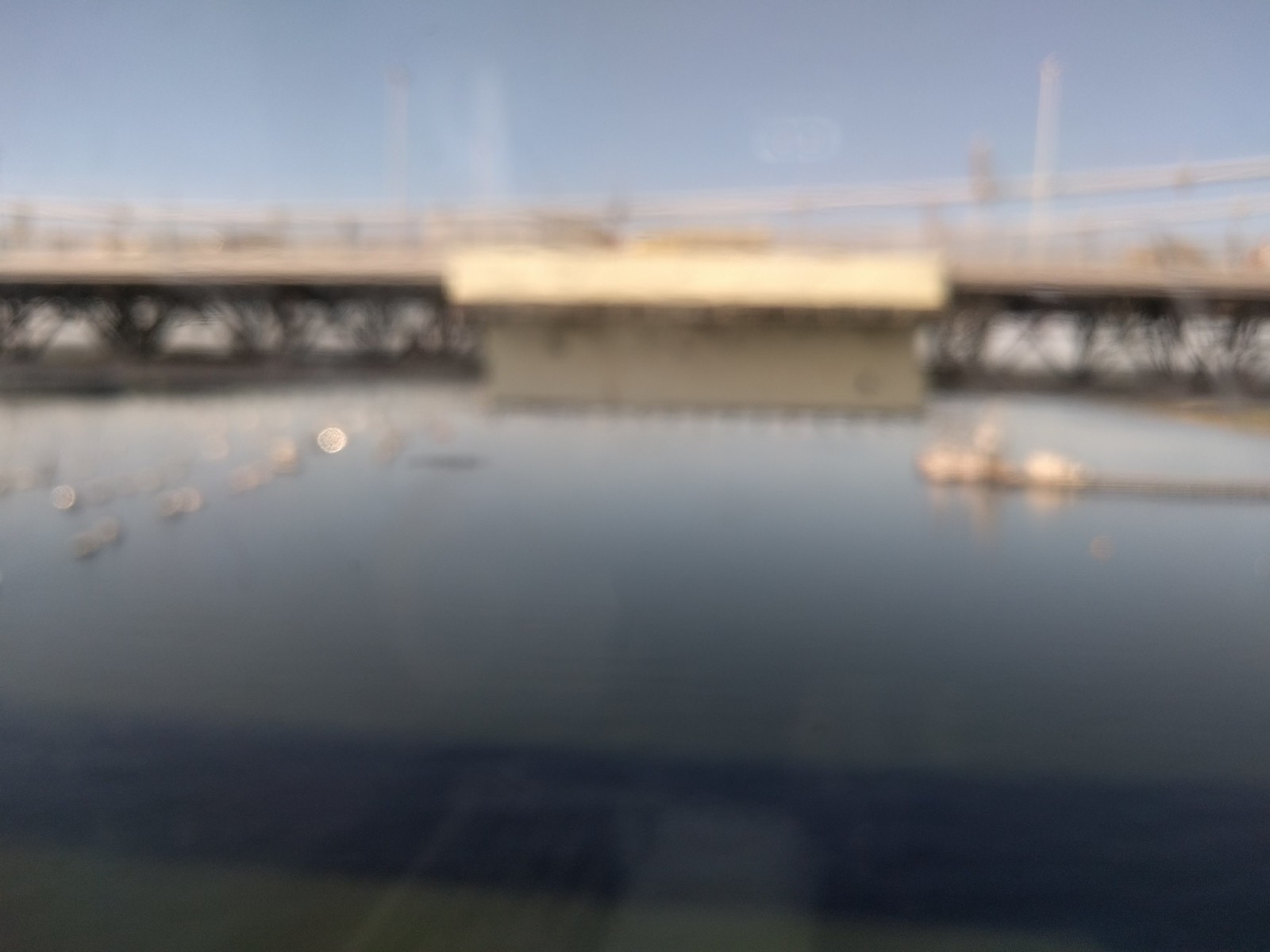A distorted photograph, likely taken through a window or glass surface, captures a scene with a discernible yet blurry reflection in the foreground. The lower portion reveals a body of water marked by faint ripples indicative of gentle waves. In the midsection, there is the faint outline of a bridge, characterized by its dark support beams arranged in an x-shaped pattern and a lighter-colored upper structure. The background shows a bluish-gray sky, and nestled in front of the bridge is a rectangular building with a light-colored façade and roof.